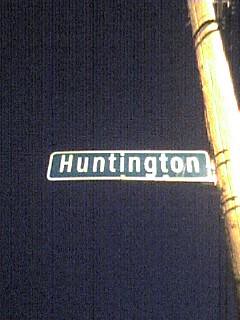This photograph captures a dark green, rectangular street sign with the name "Huntington" displayed in stark white letters. The sign is affixed to a cylindrical wooden pole situated on the right side of the image, which features band-like carvings. The scene is set against a deep, dark blue night sky devoid of stars or clouds. Both the street sign and the pole are well-illuminated, suggesting the presence of a nearby light source.